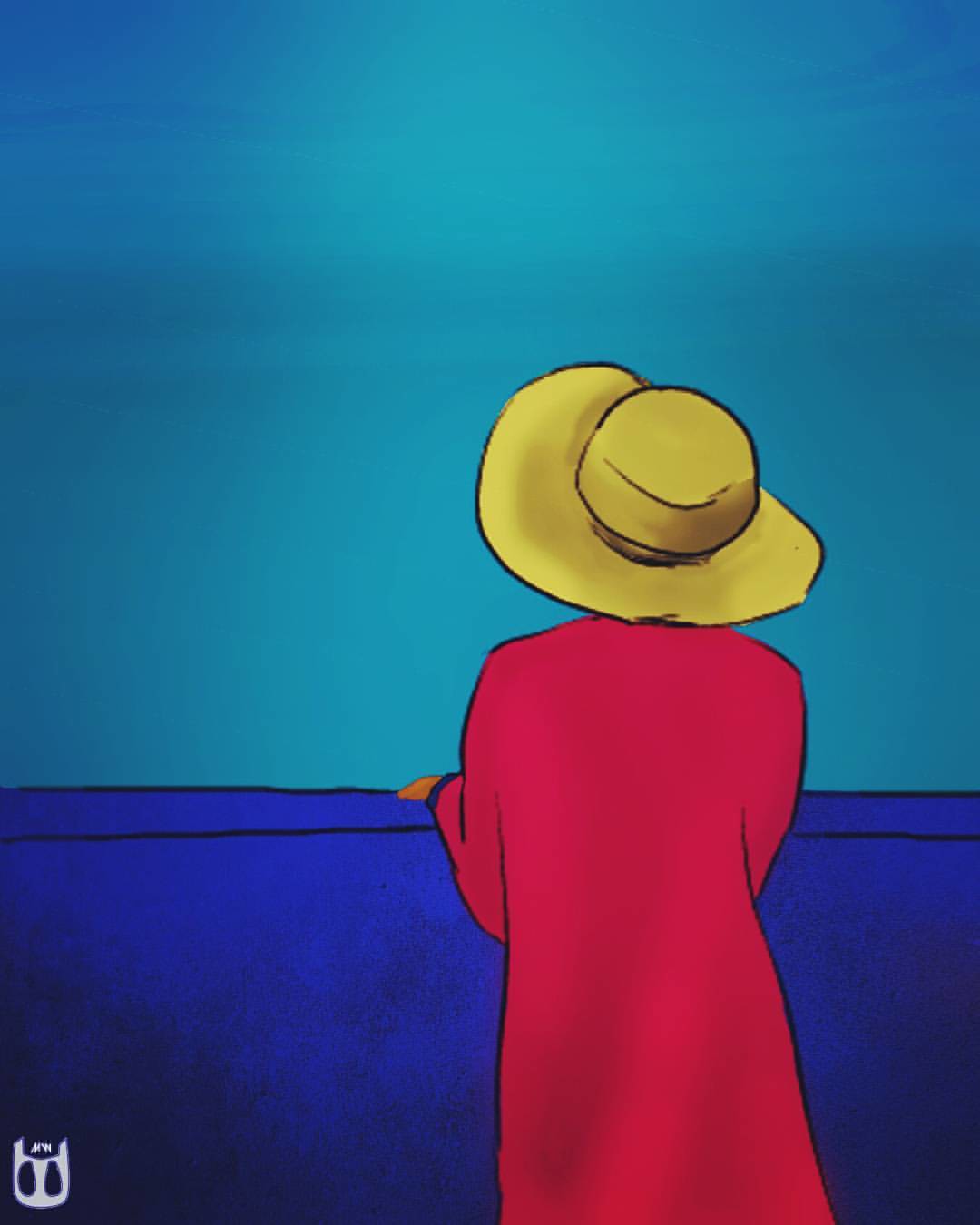In this artwork, we observe the back of a woman standing at a low, royal blue wall. The wall reaches up to about mid-torso and she rests her hands idly on top of it as she looks out into the distance. The woman is dressed in a vibrant red coat or dress with long sleeves, and wearing a pale yellow, floppy sun hat. Her skin is fair, and only her left arm and hand are visible. She appears to be gazing into the light blue sky, with a contemplative posture, leaning slightly on one hip and keeping her elbows tucked in close to her body.